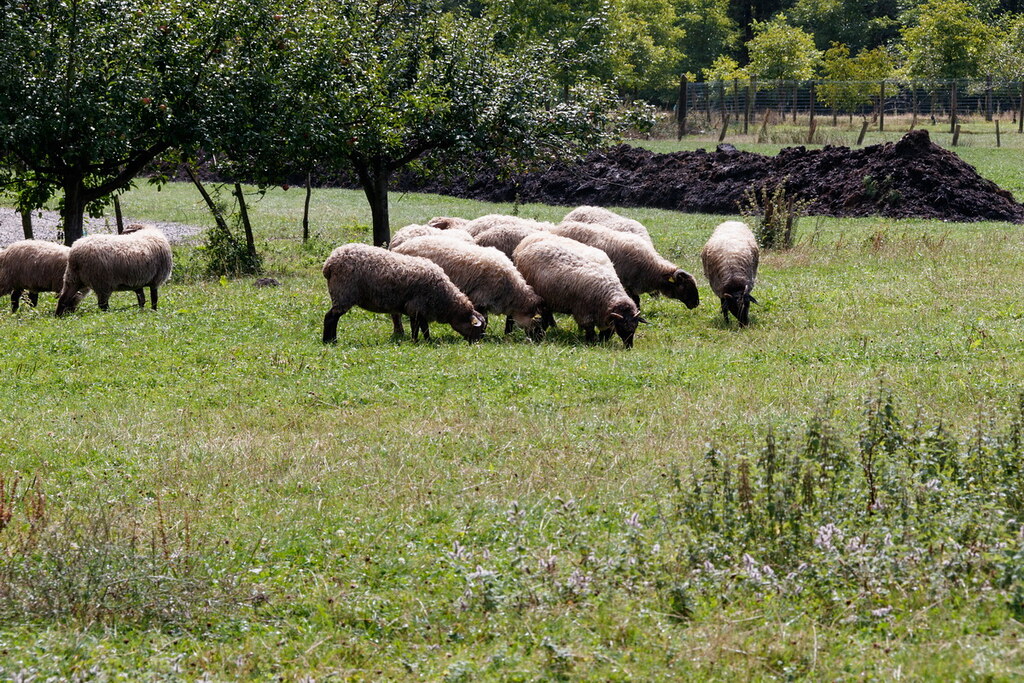In this daylight photograph, a field of lush green grass is dotted with a group of woolly sheep grazing peacefully. In the foreground, two sheep on the left side munch on the grass, while a clustered group of about eight sheep is seen a bit further to the right, all with their heads down, engrossed in their meal. The sheep have black heads and thick, off-white woolly bodies, some appearing to be in shadow or perhaps a bit dirty on their bottom halves. The field’s greenery includes taller weeds and small flowers that add to the natural scenery. In the background, a row of trees provides a scenic backdrop, with their green leaves indicating warmer weather. Further beyond the trees is what appears to be a line of black dirt or a fence blending into the background, adding depth to the pastoral setting.